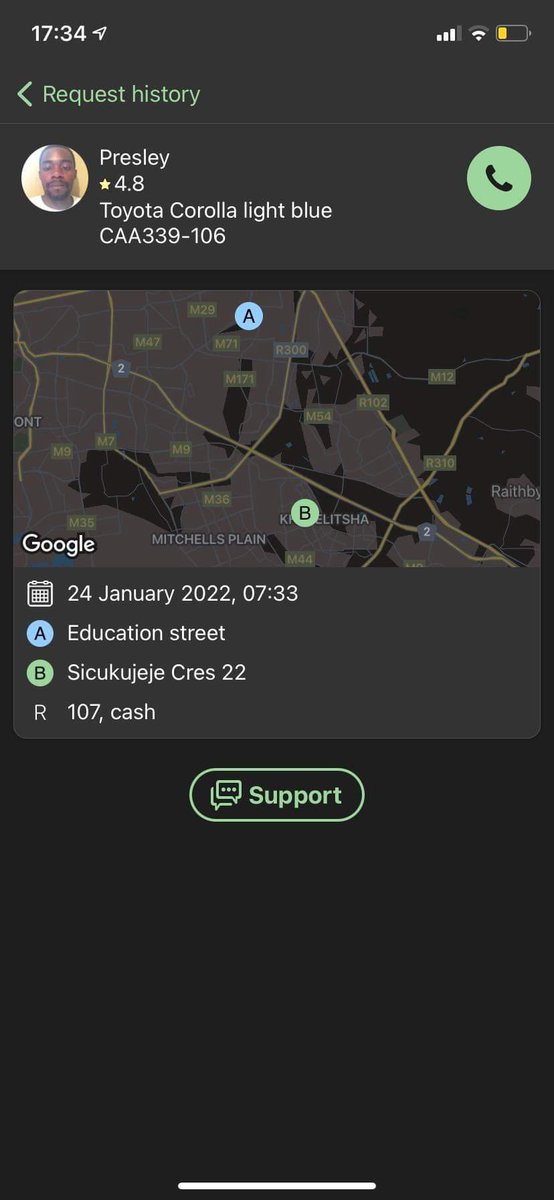The image appears to be a screenshot from a mobile phone, depicting a ride-sharing app interface on a dark background. Positioned in the upper left corner is the text "Request History." Below this text is a profile picture of an African American individual named Presley, who has a rating of 4.8 stars. Additionally, the details indicate that Presley drives a light blue Toyota Corolla, with the license plate CAA339-106. To the right of this information is a green call icon.

Beneath Presley's profile is a map set against a gray background, featuring light yellow lines that indicate streets. The map displays two marked locations: a blue circle labeled "A" at the top and a green circle labeled "B" at the bottom. The name "Google" is visible in the bottom left corner of the map. Below the map, the date "24 January 2022" and the time "7:33" are noted. The "A" location is identified as "Education Street," while the "B" location is named "SICU KU Juju Crest 22."

At the bottom of the screenshot is a support button, which features an icon with two conversation bubbles alongside the word "Support."